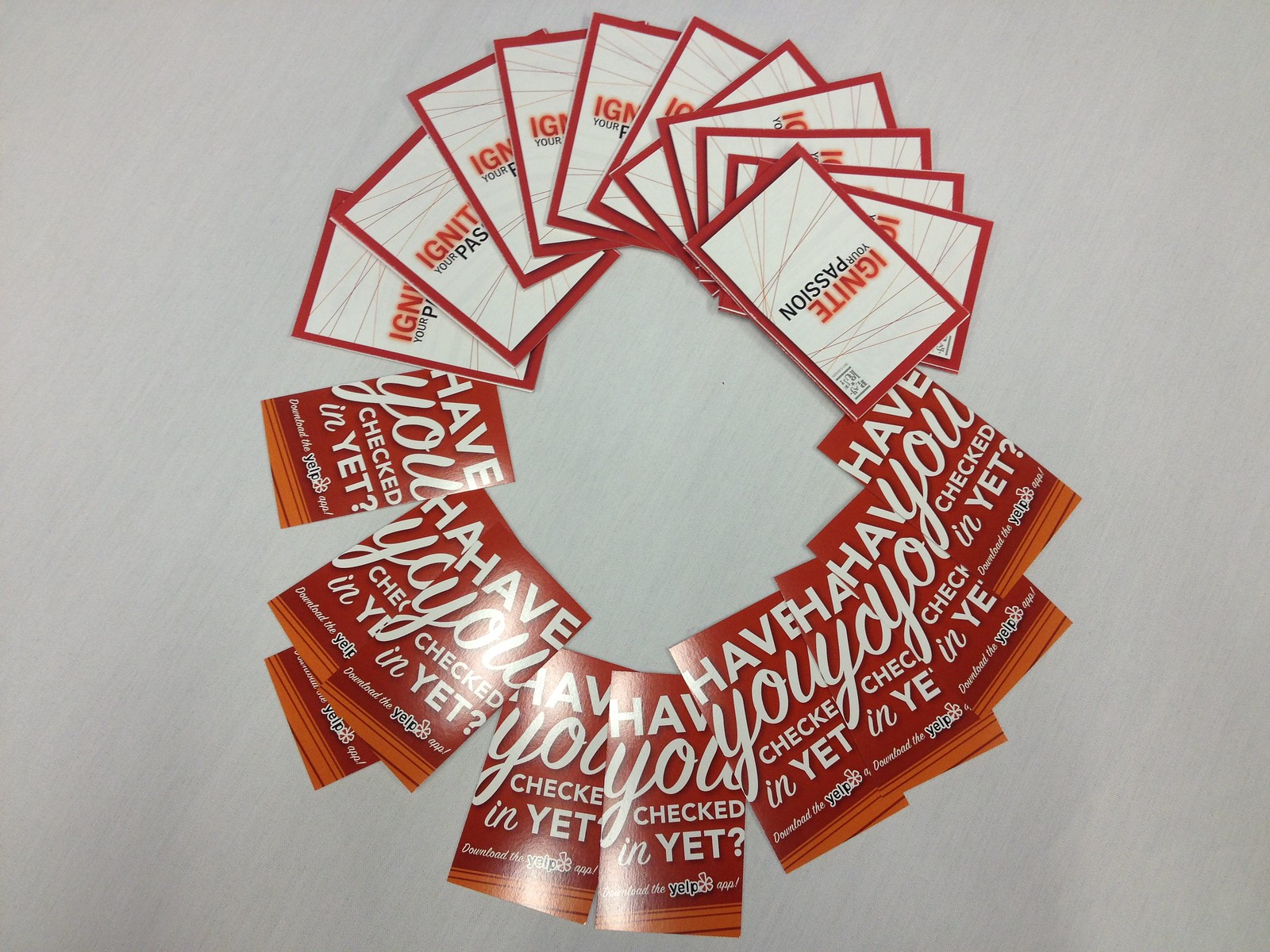A circle of cards is meticulously arranged on a plain gray surface in the middle of the image. There are two distinct types of cards forming this circular pattern. The top half of the circle features white cards with a bold red border. These cards display the phrase "IGNITE" in large red letters, followed by "your PASSION" in smaller black letters. The bottom half of the circle is made up of red and orange cards with white text that reads "Have you checked in yet?" Below this text, there is a less legible line and the recognizable Yelp logo, indicating these cards likely serve as a promotional tool for Yelp. The cards are fanned out from left to right in half-circles both on the top and bottom sections, creating a wreath-like arrangement that fills the center of the image.